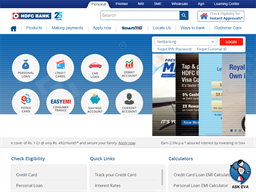This image appears to be a screenshot of a financial or banking website's homepage. The page itself is somewhat unclear due to the small and zoomed-out nature of the image. 

- **Top Section:** A blue banner runs across the top of the image. One option on the banner has been selected; it features a white tab with blurred text that could resemble the words "hobo bank," though the exact text is hard to make out. There are six additional white tabs along the banner.
- **Search Bar:** To the right of the banner is a search bar, accompanied by a blue search icon.
- **Main Banner:** Below the top section is another banner displaying an image of a red-roofed house with a blue frame. This section contains some text within a box.
- **Navigation Options:** Below the main banner is a navigation menu featuring options like a blue home icon, "Products," "Making Payments," "Apply Now," and possibly "Customer Care," though the last few options are difficult to read.
- **Feature Section:** Beneath the navigation, there is a blue background with eight circles, each containing an icon and text:
  1. A blue sack of money
  2. Possibly a wallet
  3. A red car
  4. An unclear icon
  5. A Venn diagram-like icon with a red and blue circle and dollar signs
  6. The word "Easy"
  7. A blue piggy bank with a gold coin
  8. A black silhouette
  
- **Additional Search Bar:** To the right, there is another search bar with a red search button.
- **Informational Slides:** Four overlapping slides provide some kind of information, housed in a gray banner with some text.
- **Columns Section:** Below the slides are three columns, each with a blue title:
  1. Potentially titled "Check Eligibility"
  2. "Quick Links"
  3. Possibly "Calculations"
  
Each column has two visible lines of text, but they are too small to be legible.
  
- **Icon in the Corner:** There is an icon in the bottom right corner that looks like a circle with a blue background and a silhouette of a woman or robot. Below this icon, it says "Ask Ava."

Overall, the screenshot appears to offer various navigational and informational sections typical of a financial institution's website, though the fine details are challenging to discern due to the image quality.